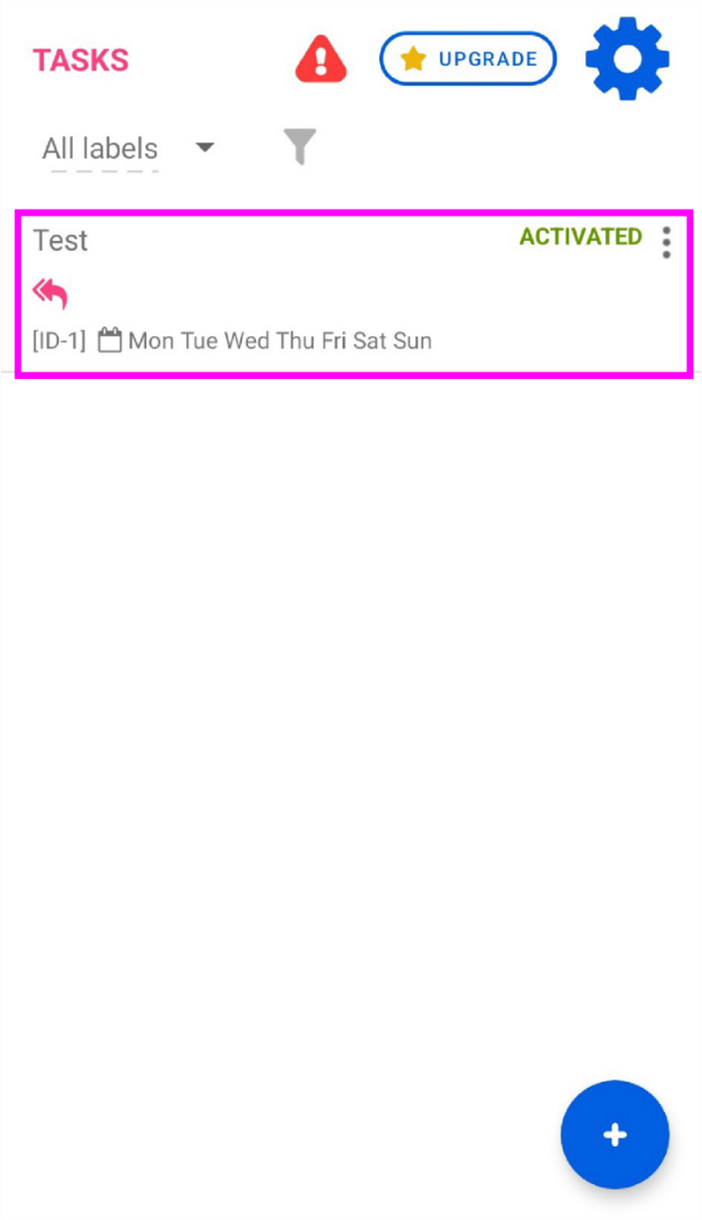This is a detailed screenshot taken from a phone, displaying a task management application with a clean white background. 

- **Upper Left Corner:**
  - The word "TASKS" is prominently displayed in uppercase pink font.

- **Upper Center:**
  - A red triangle with a white exclamation mark inside, signaling an alert or notification.
  - Next to the triangle is a gold star, likely indicating a feature or highlighted task.
  - Beside the star is the word "UPGRADE" in uppercase blue font, encircled in a blue outline.

- **Upper Right Corner:**
  - A blue settings icon.

- **Below "TASKS":**
  - A pull-down menu labeled "ALL LABELS".
  - To the right of the menu is a gray funnel icon, suggesting filter options.

- **Below "ALL LABELS":**
  - The text "TEST" appears, followed by "ACTIVATED" in uppercase olive green font.
  - To the right of "ACTIVATED" are three vertical dots, likely for additional options.

- **Below "TEST":**
  - A pink back arrow.
  - The identifier "ID-1" in brackets.
  - A small calendar icon followed by the days of the week: Monday, Tuesday, Wednesday, Thursday, Friday, Saturday, Sunday.
  - This whole "TEST" area is highlighted with a pink box outline.

- **Bottom Right Corner:**
  - A blue circle with a white plus sign in the center, suggesting an option to add a new task.